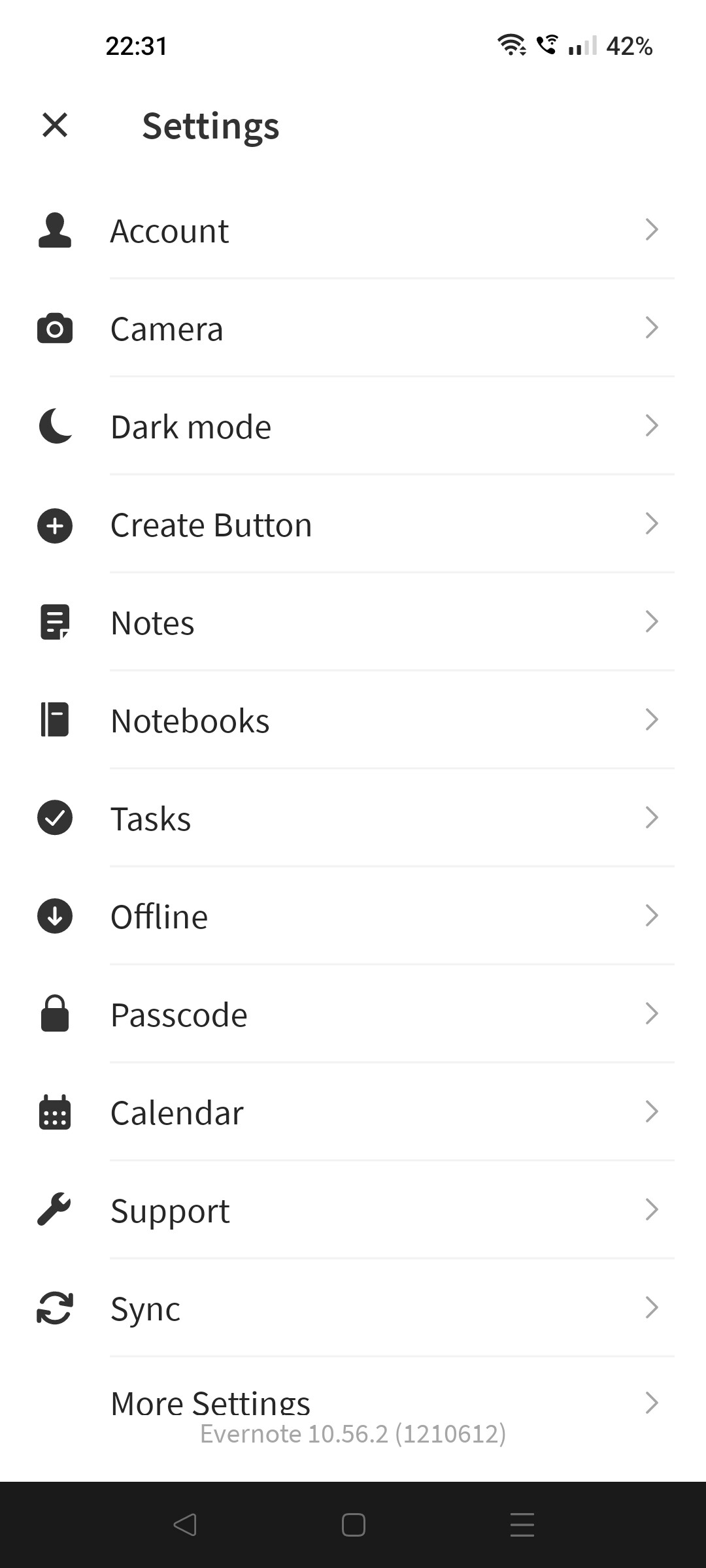In the top left corner of the screen, the time is displayed as 22:31. The top right corner shows several icons: a Wi-Fi signal bar, a phone icon, a cell phone signal indicator with two out of four bars filled, and a battery icon showing 42% charge. Below these icons, the header reads "Settings" with an "X" icon beside it to close the menu.

The main section of the screen displays various settings categories listed vertically. Each category has an icon on the left and its label on the right, separated by thin gray lines. The categories are:

1. Account
2. Camera
3. Dark Mode
4. Create Button
5. Notes
6. Notebooks
7. Tasks
8. Offline
9. Passcode
10. Calendar
11. Support
12. Sync

To the right of each category label, a small gray arrow points to the right, indicating that they can be expanded or selected for more options.

At the very bottom of the screen, there is a black background containing three navigation icons: a left-pointing triangle on the left, a square in the middle, and three small horizontal gray lines on the right.